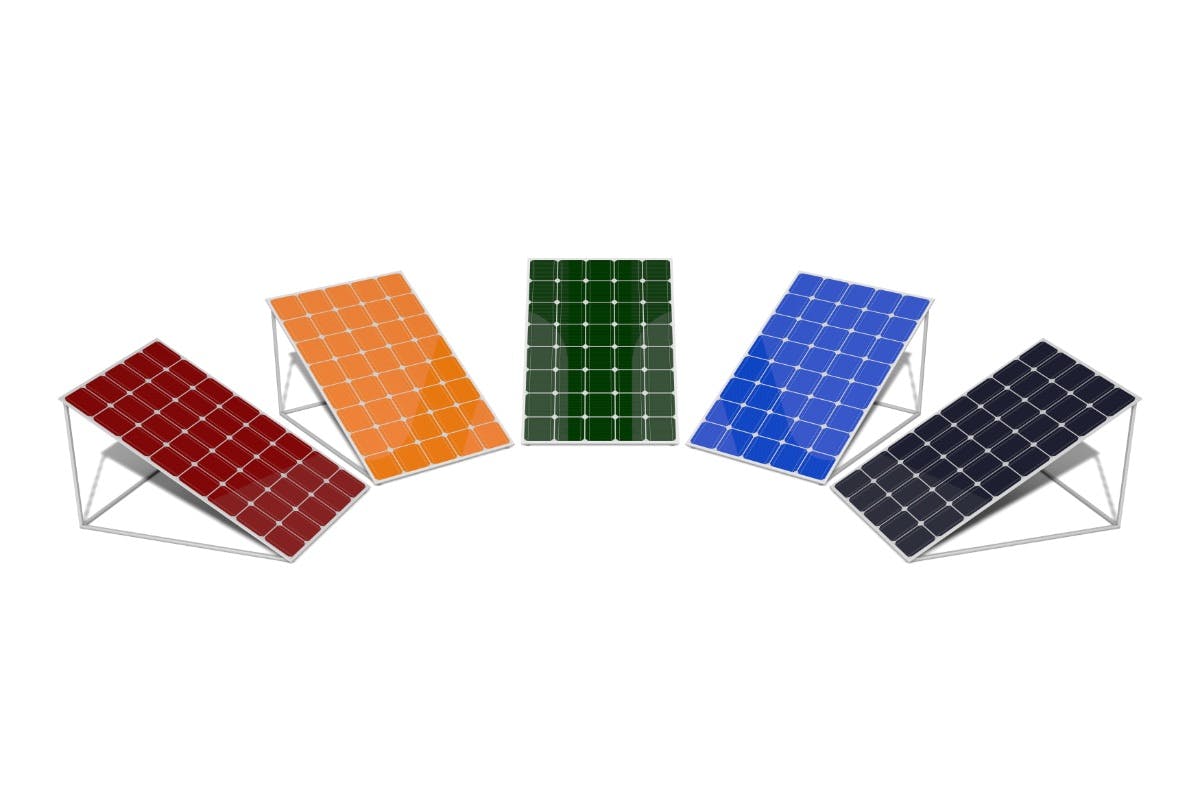The image depicts a set of five rectangular objects that resemble solar panels, each mounted on a white block stand. The panels are arranged in a fan-like, semicircular formation, creating a slight arc or frown shape. These panels are divided into a grid of small squares by white lines. From left to right, the colors of the panels are maroon (red), orange (yellow), green, blue, and a very dark blue or black. All panels appear to be the same size and are tilted at approximately a 45-degree angle, facing upwards. The distinct colors and orderly separation by lines give the array a striking and organized appearance within the white, borderless background.